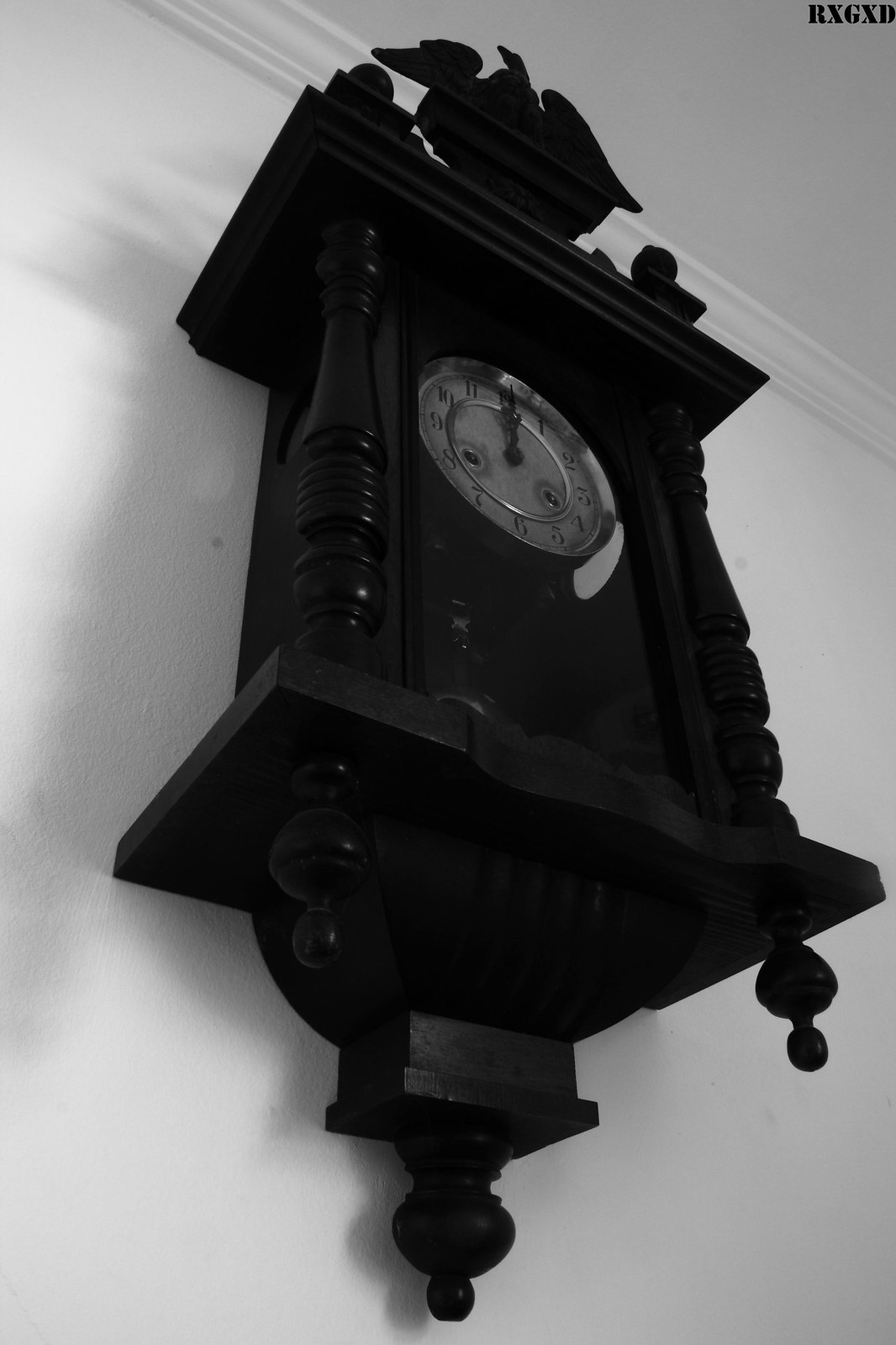A black and white vertical photograph captures an upward perspective view, emphasizing its dramatic composition. Dominating the upper portion of the image is a traditional, old-fashioned cuckoo clock, rendered in a deep espresso brown hue. The clock is richly detailed, featuring ornamental posts on its sides and an intricately carved backing that descends with graceful curves and bulges. Atop this exquisite structure, a decorative bird perches, adding an extra touch of vintage charm. The clock face itself is a striking silver, with hands indicating twelve o'clock, lending a static sense of time. The ceiling above, along with a pristine strip of white crown molding and an adjoining wall, forms the backdrop, providing sharp contrasts that highlight the clock's elaborate craftsmanship. The photograph, while contemporary, utilizes monochrome tones to evoke a timeless, nostalgic atmosphere.